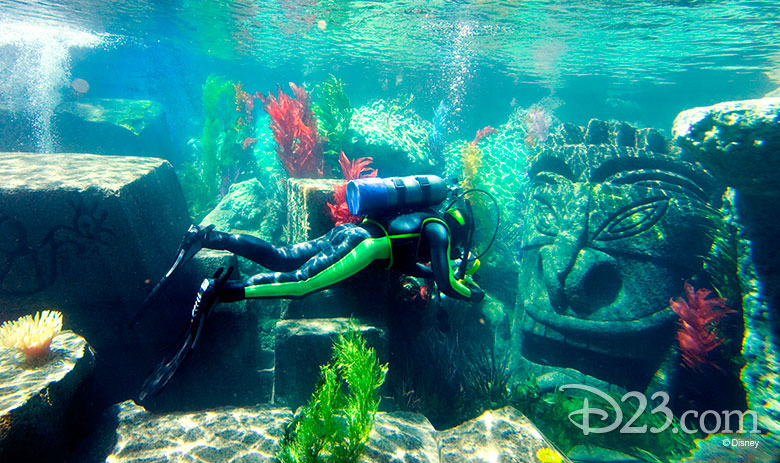The vibrant underwater scene is vividly lit, showcasing a striking array of colors dominated by aqua and teal hues, with the sun's radiance shimmering on the water's surface above. A diver, clad in a distinctive blue and green neon wetsuit complete with a tank and flippers, hovers prominently in the foreground. Surrounding them are remnants of submerged ruins, including a row of imposing stone blocks, each approximately six feet in height and width. Directly to the right of the diver's head is an intimidating, Mesoamerican-styled stone carving, featuring a large toothy mouth and frowny eyes. Green aquatic plants sprout from the seabed immediately in front of the diver, adding to the lifelike scenery. The depth of the setting is relatively shallow, between 10 to 20 feet, revealing a man-made stage depicting ancient ruins, possibly crafted by Disney as suggested by the D23.com logo in the lower right corner.